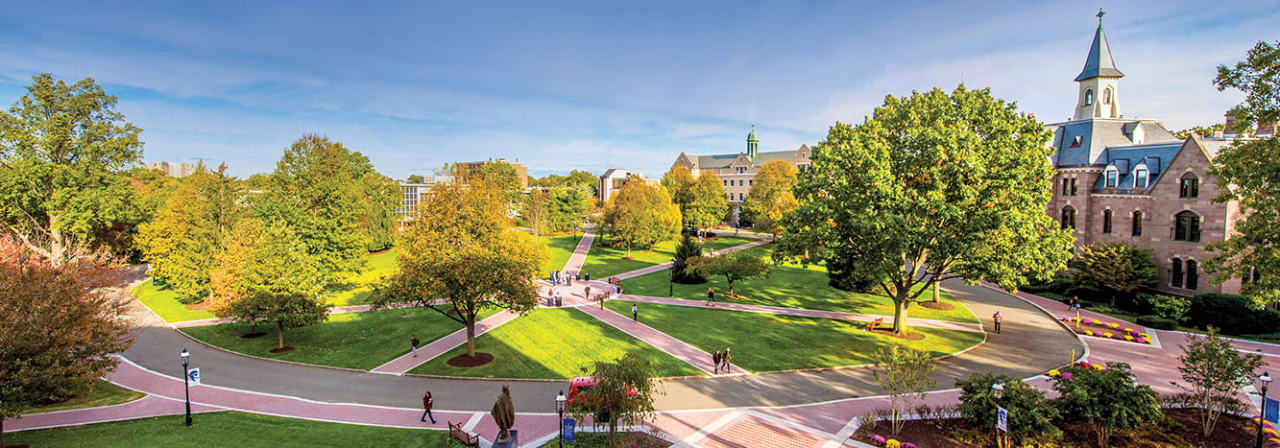This wide-angle aerial photograph, taken in bright sunlight, captures a vibrant, perhaps autumn, scene dominated by a large traffic circle or quad, central to a college-university campus. At the heart of the image is a central circular area with radiating brick sidewalks forming spokes that connect to an outer circle. This central quad is lush with various shades of green and hints of fall colors, including tall trees with orangey and green foliage, and meticulously manicured areas with flowers planted in soil. There is a noticeable statue near the middle of the traffic circle among the greenery. 

To the far right, a prominent brick building resembling a university structure, complete with three levels of windows and a chapel-like section topped with a cross, is visible. Surrounding this main building are other less distinct structures, partly obscured by trees. The scene is bustling with life, as small-scale figures of people can be seen milling about the quad and walking along the sidewalks. The setting is idyllic under a blue sky adorned with high, wispy white clouds, casting distinct highlights and shadows across the landscape.